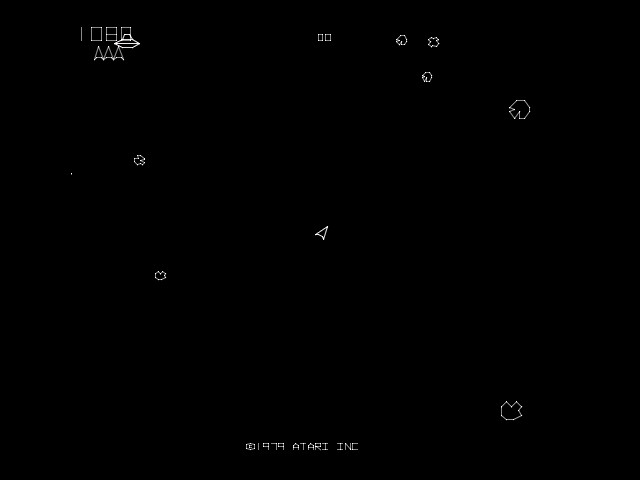The image features a classic Atari game displayed on a square screen with a completely black background and white, pixelated game elements. Dominating the center of the screen is a prominent navigational triangle, likely representing the player's controlled entity. Scattered across the screen are various game pieces, including round objects and uniquely shaped elements. Notably, in the bottom right-hand corner, there is a distinctive piece resembling an upside-down mushroom. Higher up, along the right edge of the screen, another similar mushroom-like shape appears, oriented differently. These elements, combined with other smaller round pieces, contribute to the classic, nostalgic feel of the game.